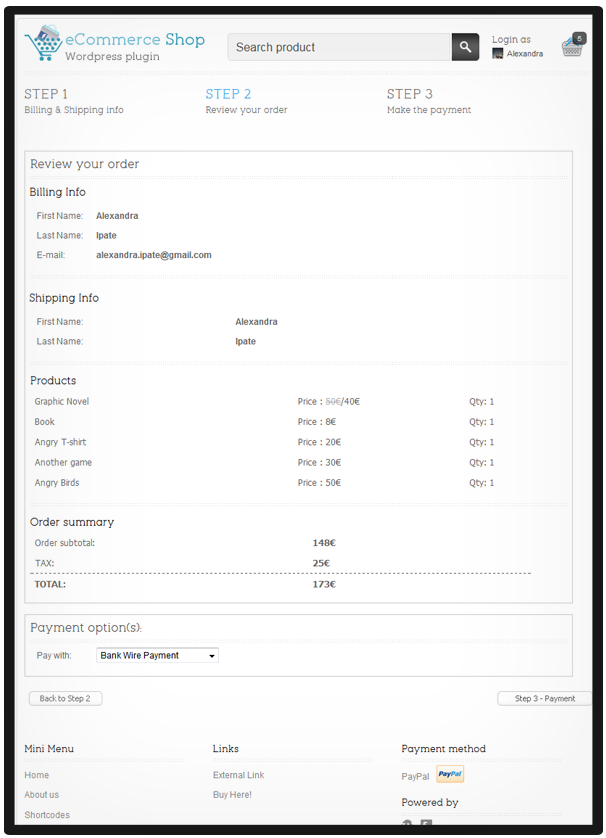The screenshot features a light gray background and prominently displays a company logo in the upper left-hand corner. Next to the logo, in bold blue text, is the title "eCommerce Shop," followed by "WordPress Plugin" in gray text just below it. To the right of these words is a search bar, featuring a black square with a white magnifying glass icon on its right side. Further to the right is an option labeled "Login As."

Horizontally aligned below this header section are three steps denoted as "Step 1," "Step 2," and "Step 3" with accompanying descriptions beneath each step, all in gray except for "Step 2," which is highlighted in blue to indicate the current stage.

The main content area features a large square box. In the upper left-hand corner of this box, it reads "Review Your Order." Below that are sections labeled "Billing Info," "Shipping Info," "Products," "Order Summary," and "Total."

Towards the bottom of the main content area, there is a rectangular section containing payment options. It is labeled with "Pay With" and features a dropdown box that currently displays "Bank Wire Payment" in bold text. Adjacent to this section is a button on the left side.

At the bottom of the screenshot, there are three columns. The left column is titled "Main Menu," the middle column is titled "Links," and the right column is titled "Payment Method." Just above these columns, beneath the payment options, is another button on the right side that partially reads "Payment."